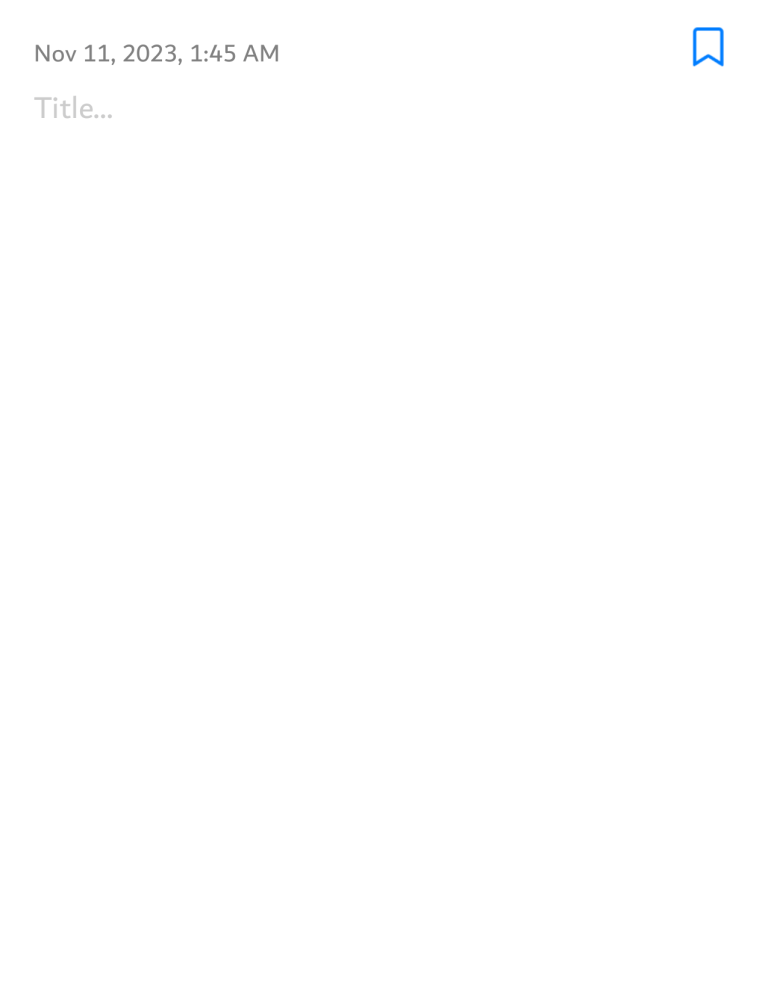Screenshot of an empty field with the timestamp "NOV 11, 2023, 1:45 AM" prominently displayed in gray text at the top left corner. Below the timestamp, in a lighter gray and larger font, is the word "title..." On the right side of the image, there is a blue banner icon. The background of the image is predominantly white, and the remaining portion of the image is blank, highlighting the absence of additional content or graphics.